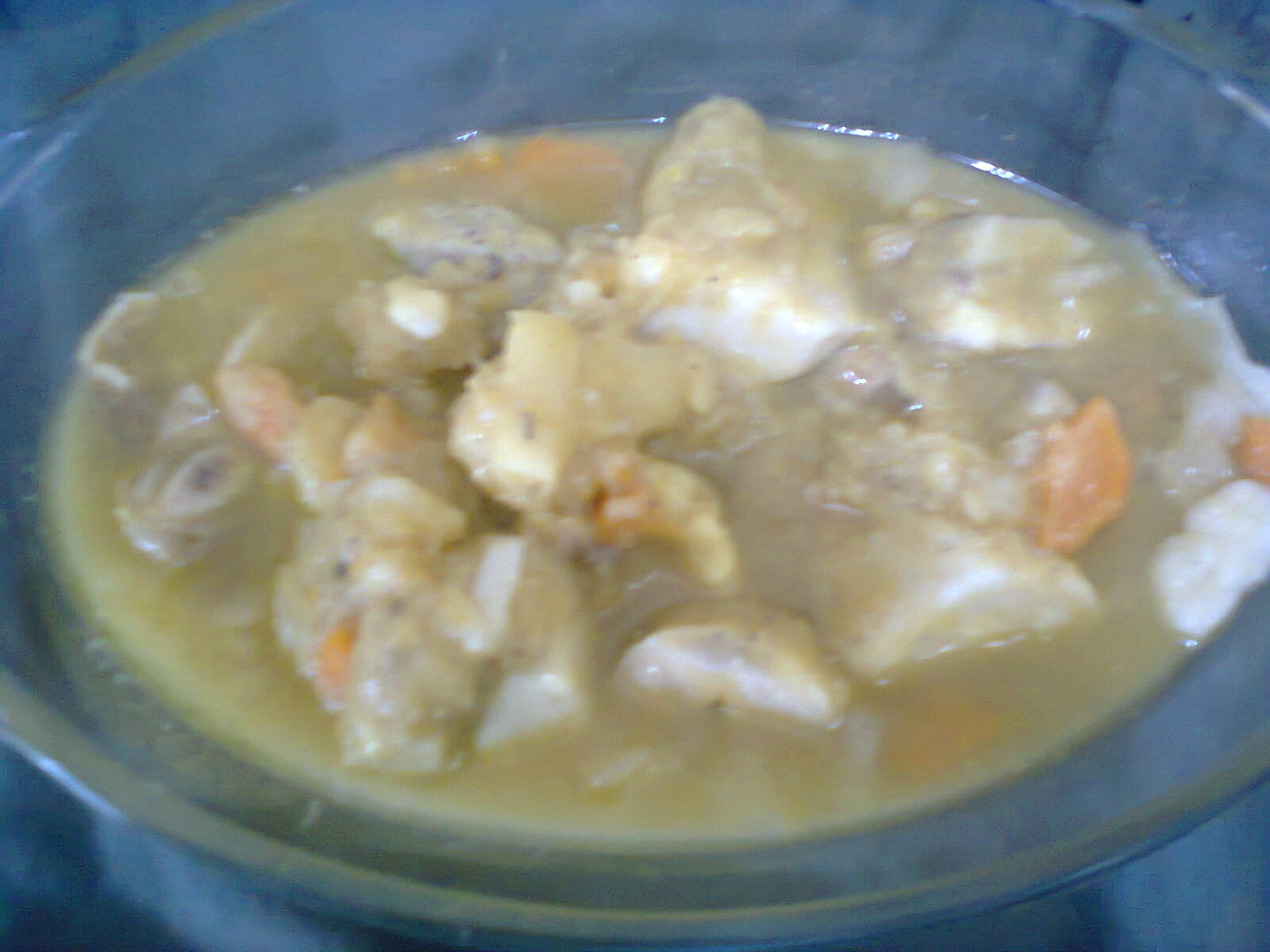This is a horizontally aligned, somewhat blurry photograph of a close-up, clear glass bowl containing a hearty stew. The bowl, resting on a blue quilted fabric—likely a tablecloth or placemat—allows you to see the table through it due to its transparent nature. The stew inside appears to be a rich, medium to light brown broth, hosting a medley of ingredients. Dominating the stew are chunks of meat, potentially chicken given its light color, adorned with small round, oval-shaped bones and occasional visible fat. Interspersed throughout the dish are small orange pieces that resemble cut-up carrots and an array of brown square and rectangular chunks, likely potatoes. The broth's lightness hints at a chicken stock base. Despite the image's blurriness, these elements are distributed evenly in the bowl, creating a balanced and visually appealing composition.